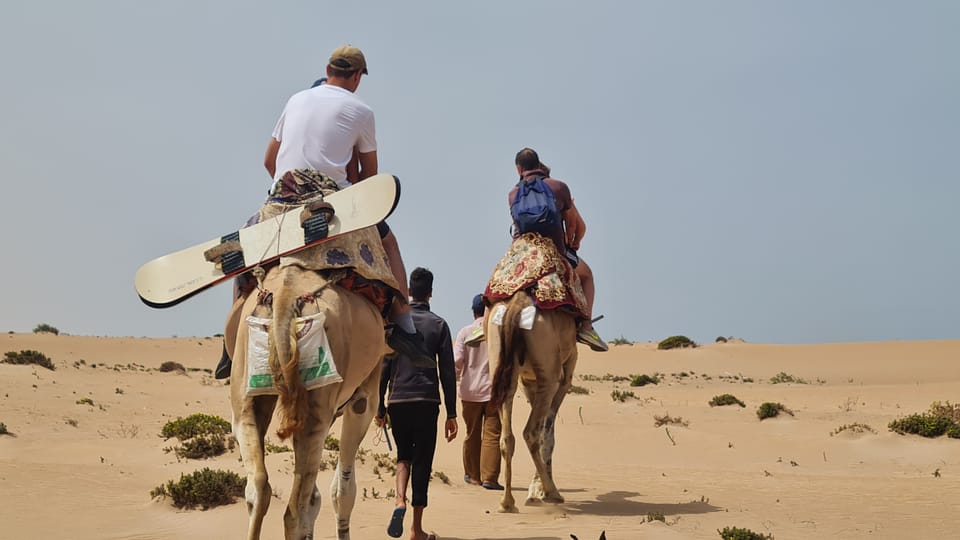In this detailed desert scene, a bright, clear sky stretches above a sandy landscape dotted with small clusters of arid bushes. Dominating the scene are two camels, each adorned with flower-themed throws and carrying two riders. The left camel has a snowboard strapped to its saddle, and its riders include one person wearing a white t-shirt and a brown hat. On the right camel, the rear rider sports a blue backpack while the other wears a brown shirt and shorts, with their legs exposed. Walking beside the camels are two men, adding a sense of movement to the photograph. The vibrant sunlight highlights every detail, making the image crisp and clear.